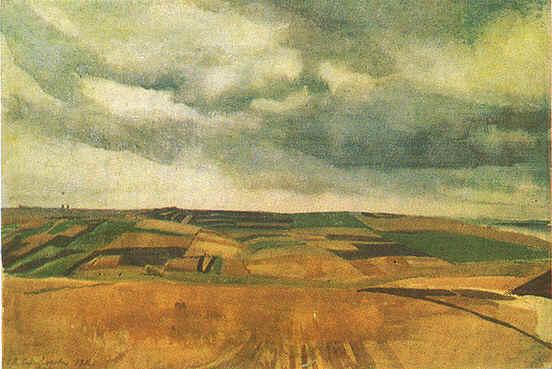This image is a detailed painting of a farmland landscape. The vantage point appears to be from the top of a yellowish-tan hill, situated in the foreground. Beneath the hill sprawls a vast array of fields, each distinctly colored—greens, various shades of browns, grays, and even a black plot. These fields are generally square or rectangular and extend far into the distance, with a total of approximately 15 different sections. In the background, two trees are visible, possibly near a farm structure or silos on the far left, adding depth to the scene. The expansive sky occupies the upper half of the image and is depicted with a mix of white, gray, and dark blue clouds, creating a gloomy, rain-threatening atmosphere. To the right side of the fields, the land appears to meet another type of terrain, possibly an ocean or different landscape, bringing the farmland to an end.